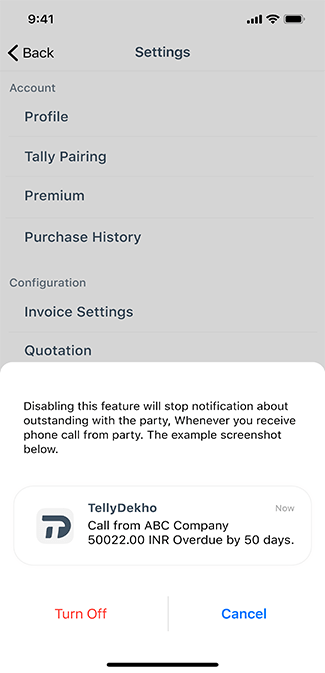The screenshot features a light gray status bar at the top displaying the time as 9:41, along with full Wi-Fi signal, and a fully charged battery icon. Below the status bar, there's a navigation bar with a back arrow pointing to the left and labeled "Back," next to the title "Settings."

Within the Settings menu, there is a list of options including: 
- Account Profile
- Tally Pairing 
- Premium 
- Purchase History 
- Configuration 
- Invoice Setting 
- Quotation

Beneath the list, the screen has a section with a white background and black text, stating: "Disabling this feature will stop notifications about outstanding amounts with the party whenever you receive a phone call from the party. See the example screenshot below."

Following this text, there's a box with a gray border containing a white background. Inside, there's a gray and dark blue logo labeled "Teledeco." The example notification within this box reads: "Now calling from ABC Company. INR 50022.00 overdue by about 50 days." Below this notification, there are two action buttons: one red button labeled "Turn Off" and one blue button labeled "Cancel."